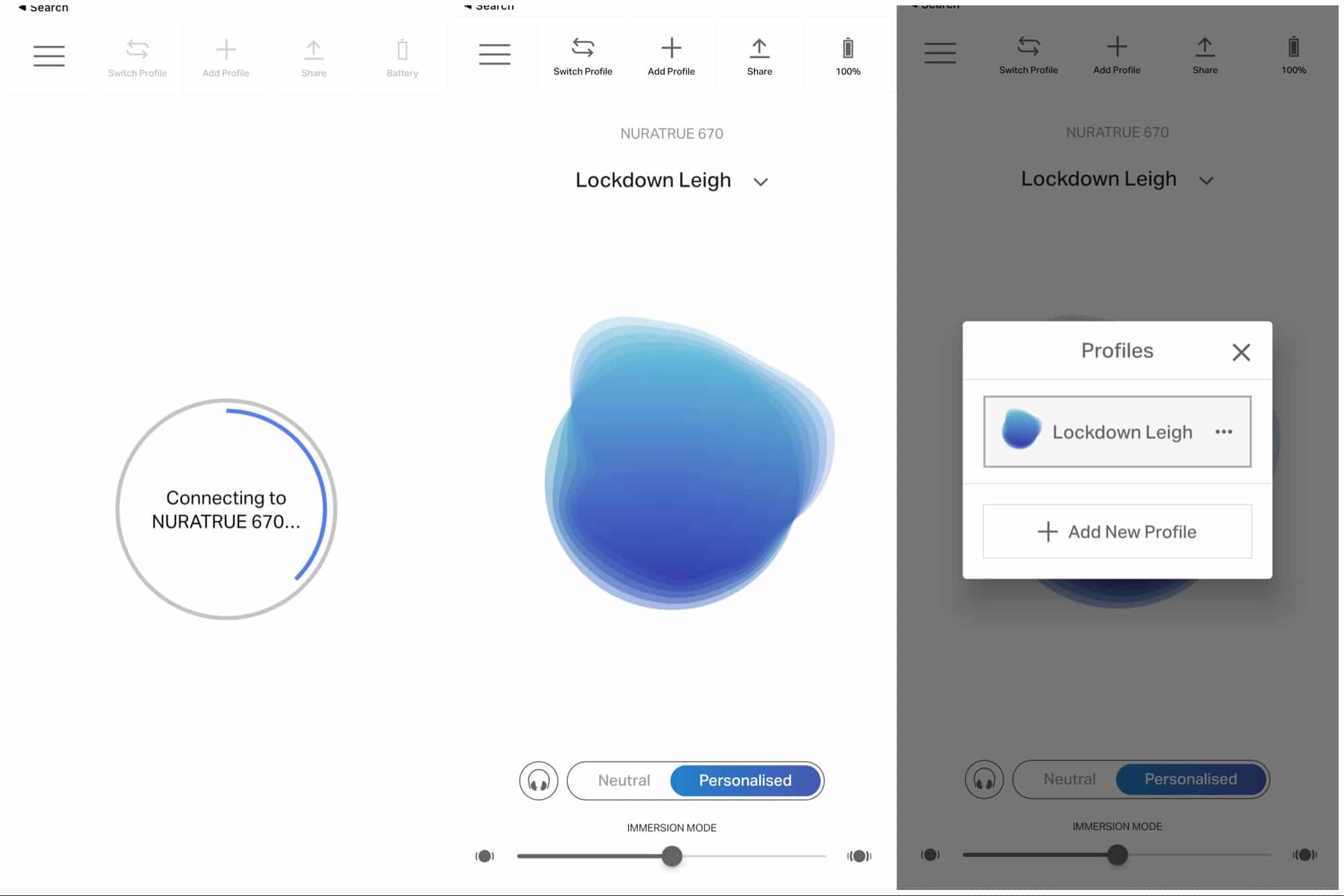The image is a composite of three side-by-side screenshots, likely taken from a mobile application. Each screenshot appears to be from an app interface, capturing different moments of interaction:

1. **First Screenshot:**
   - **Background:** White
   - **Header Icons (Left to Right):** Three horizontal lines (menu), "Switch Profile" button, "Add Profile" button, up arrow for share, and a battery icon (grayed out).
   - **Main Content:** A circular icon with the text "Connected to NUR Nature 670."

2. **Second Screenshot:**
   - **Background:** White
   - **Header Icons:** Same as the first screenshot, but the icons are darker and less transparent.
   - **Main Content:** At the bottom, the text "NUR True 670 Lockdown Li," a blue blob indicating some sort of activity or status. 
   - **Interactive Elements:**
     - A toggle button, currently switched on.
     - A "Personalize" button in blue.
     - The word "Neutral" grayed out.
     - A slide bar underneath these elements.

3. **Third Screenshot:**
   - **Background:** Gray
   - **Header Icons:** Identical to the first and second screenshots.
   - **Main Content:** Similar to the second screenshot, but with a gray background.
   - **Additional Element:** A box overlaid on top displaying "Profiles Lockdown Li," with an option to "Add New Profile."

This detailed comparison suggests that the screenshots show the app in different states or versions, possibly capturing user interactions like switching profiles or personalizing settings.